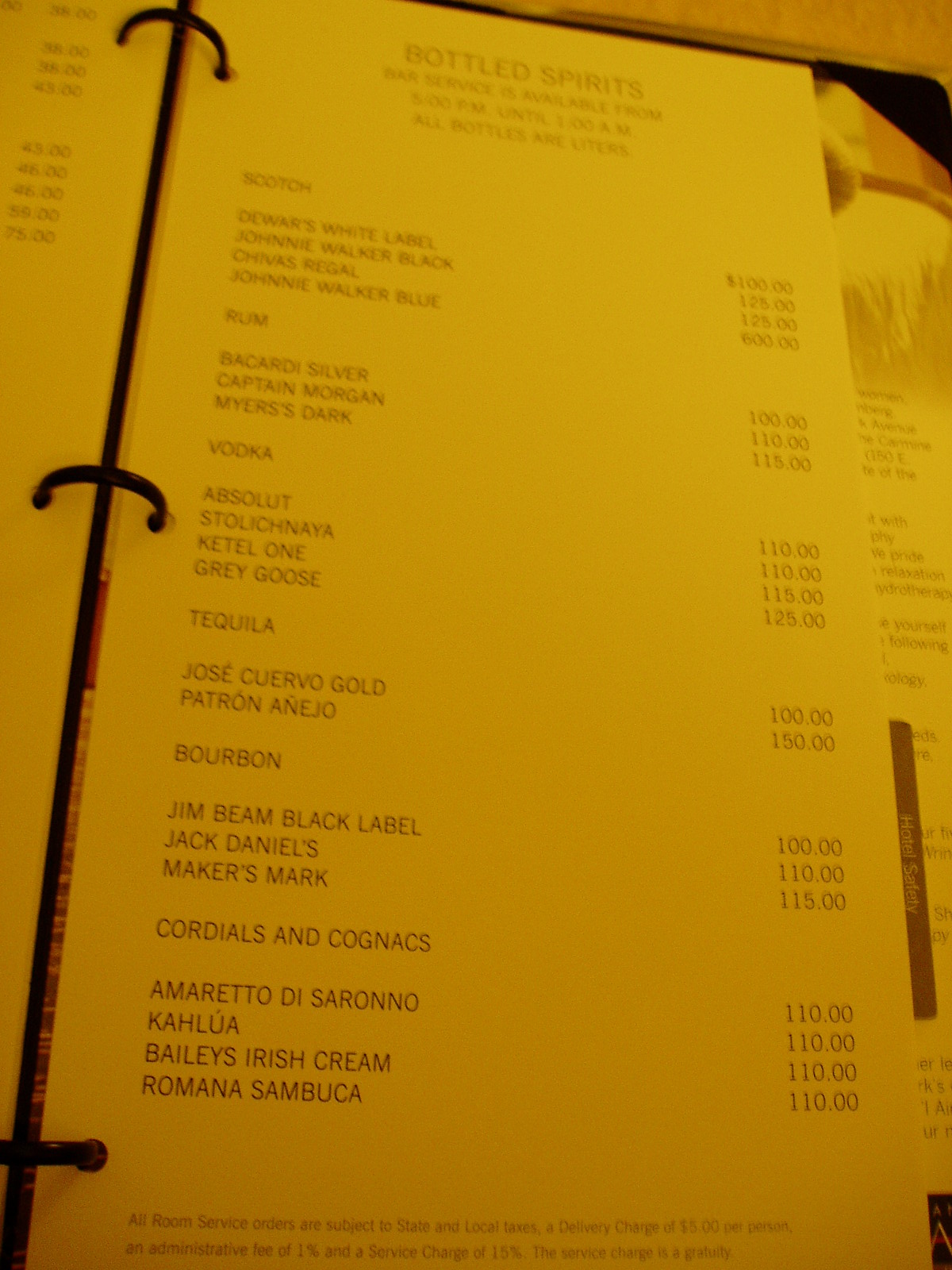The image captures a detailed page from a room service wine and spirits menu, housed within a spiral-bound notebook with three black rings. The notebook is open to a page titled "Bottled Spirits" in black text, with lighting giving the yellowed sheet an aged appearance. Beneath the title, smaller, grayish text outlines the hours of availability, from 5 p.m. to 1 a.m.

The menu is organized by types of spirits, starting with scotch, listing brands and their prices. Notable entries include Dewar's White Label priced at $100 and Johnny Walker Blue at $600. Next, the rum section features Bacardi Silver at $100, Captain Morgan, and Meyers Dark at $115.

The vodka section lists Absolut for $110, Stolichnaya, Ketel One, and Grey Goose, with Grey Goose being the most expensive at $125. Under tequila, Jose Cuervo Gold is $100, while Patron Anejo is $150. For bourbon, the list includes Jim Beam Black Label, Jack Daniels, and Maker’s Mark, ranging from $100 to $115.

The menu concludes with Cordials and Cognacs, including Amaretto di Saronno for $110, Kahlúa and Bailey’s Irish Cream at $110 each, and Romana Zambuca also priced at $110. The page, predominantly yellow with light brown print, presents a comprehensive selection of spirits available for room service.